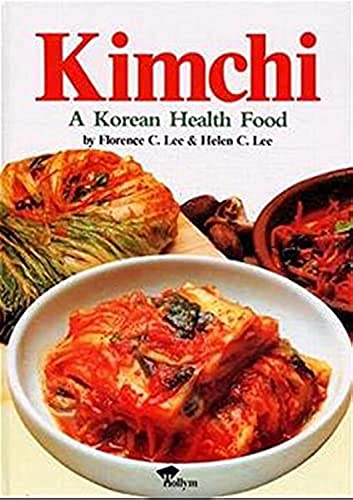The cover of the cookbook, titled "Kimchi," prominently features its name in large red letters against a white background. Below the title, in smaller black text, it reads "A Korean Health Food" by Florence C. Lee and Helen C. Lee. The center and lower portions of the cover are dominated by vibrant images of Korean dishes. The central image showcases a delicious-looking white bowl filled with spicy red kimchi noodles topped with greens, possibly spinach. To the right, there's a wooden bowl filled with red-hued food, suggesting rich spices or fermented vegetables. On the left, there's a circular piece of food, likely a fermented cabbage, resting on a wooden cutting board adorned with red streaks and specks, indicating the fermentation process. The overall composition suggests a rich, flavorful exploration of Korean cuisine.